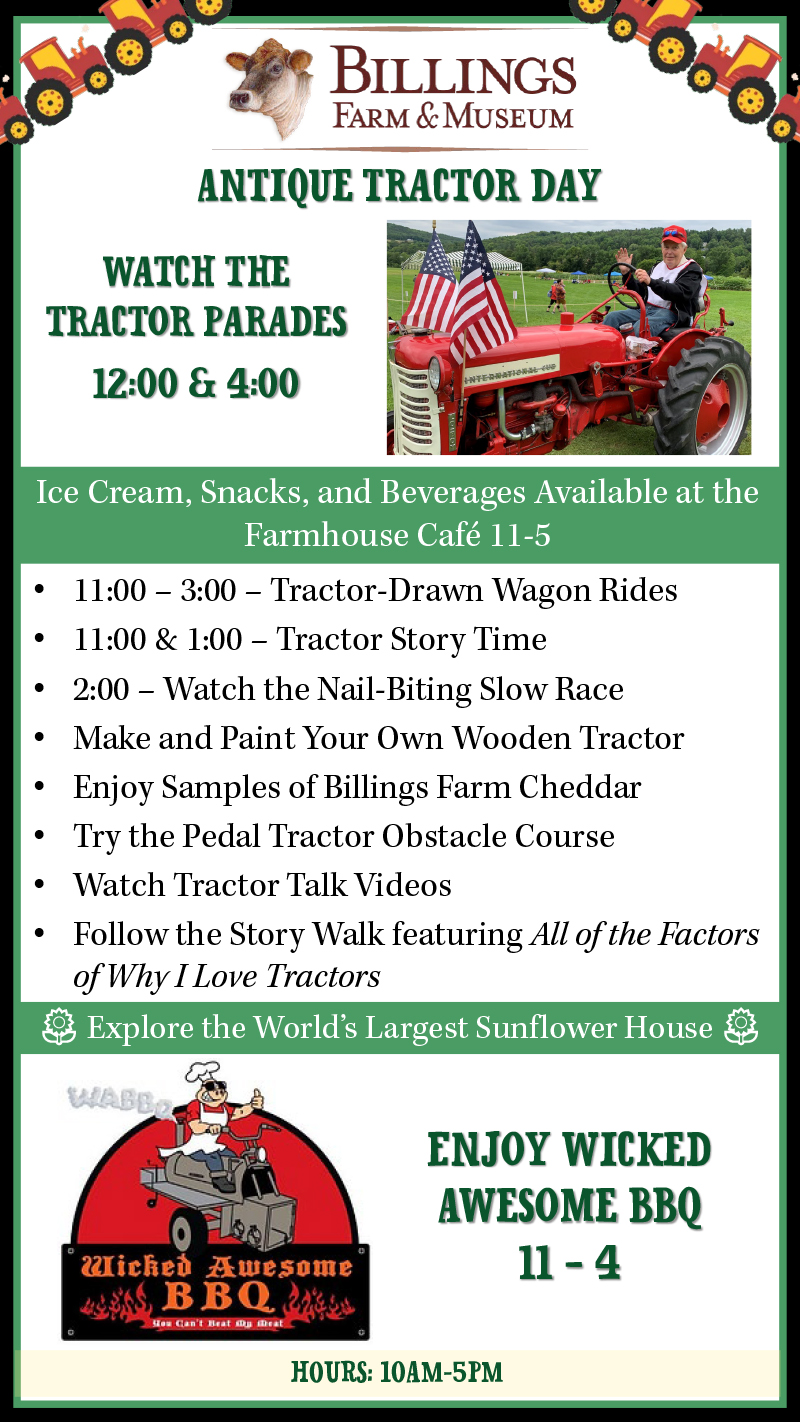This is a poster advertising Billings Farm and Museum's "Antique Tractor Day." The poster features a clean white background bordered by black and green trim. At the top, the heading "Billings Farm and Museum" is accompanied by a detailed illustration of a cow, colored gray with a brown patch on its head. Flanking this title are images of antique tractors in red and orange as corner embellishments. Below the heading, the green text "Antique Tractor Day" prominently stands out. Next to this title is a photograph of a smiling man driving a red tractor adorned with two American flags. Beside the image, the text "Watch the Tractor Parades 12 and 4 o'clock" beckons visitors to the scheduled parades. Further down, a green callout box announces, "Ice Cream, Snacks, and Beverages Available at the Farmhouse Cafe from 11 to 5." The poster also provides a detailed itinerary of the day’s events, featuring activities like Tractor John Wagon Rides and the Nail-Biting Slow Race at 2 o'clock. At the bottom, the emblem of "Wicked Awesome Barbecue" depicts a character ready to cook, highlighting one of the event's food vendors available from 11 to 4.